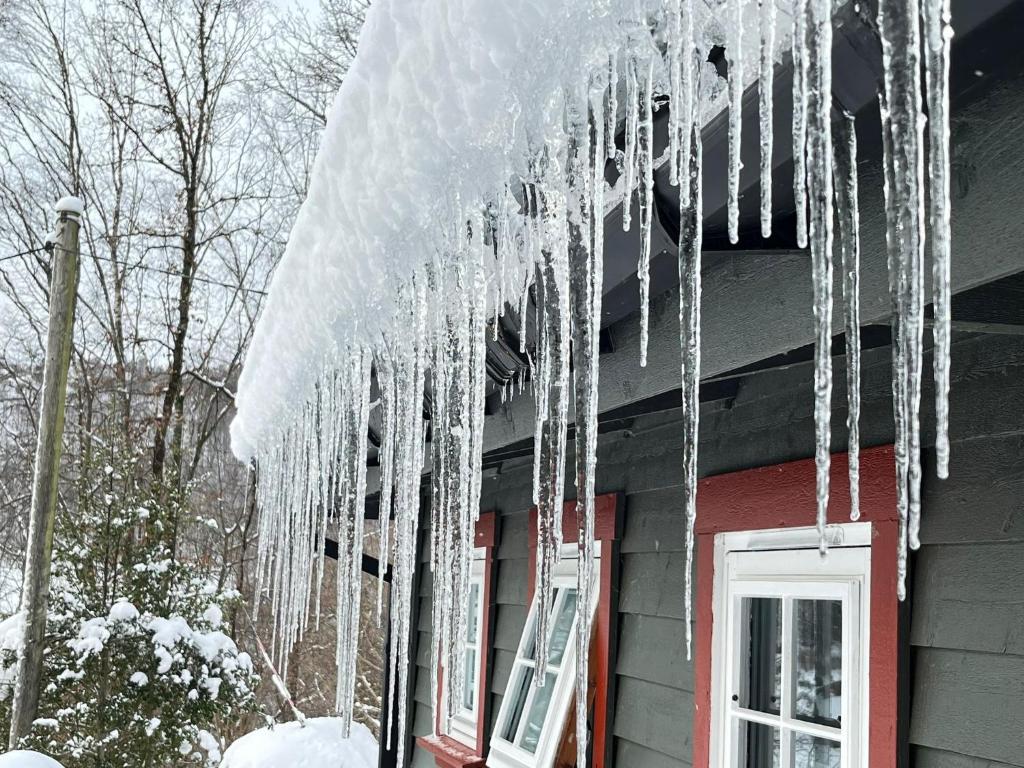The image is a color photograph in landscape orientation, capturing a winter scene of the side of a house. The focal point is a gutter along the top edge of the roof that is overflowing with ice, forming a significant white frozen mass. Numerous long, clear icicles hang from the frozen gutter, extending from the top to the bottom of the photograph. Below the icicles, the house features dark gray horizontal lap board siding, accented with brick-colored trim around the windows. There are three visible windows, framed by a white inner trim and a wider red outer frame, with the middle window slightly propped open. On the left side of the image, a snowy landscape is visible, including short shrubs near the bottom left corner and tall, snow-covered dead trees. Additionally, a snow-covered electrical pole extends into the scene with a wire leading to the house. The roof is topped with snow, and the sunlight creates a slight overcast effect due to the snow. The overall style of the photograph is a detailed and realistic representation of a typical winter day.